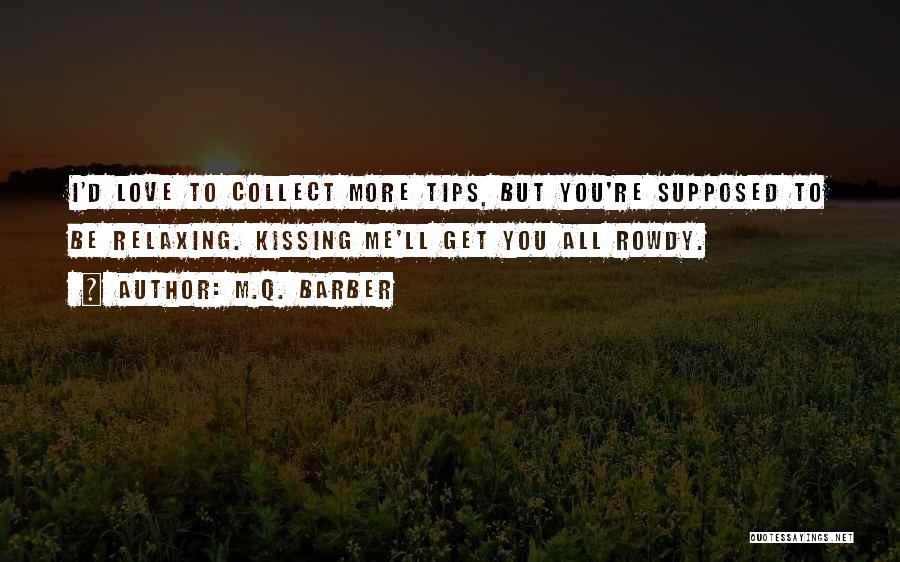In the image, a shadow-filled meadow with tall grass, bushes, and scattered little flowers is depicted against a dark, faded background. Near the horizon on the left, a sliver of the sun peeks through, suggesting either a sunset or sunrise, with a row of distant trees silhouetted against a dim sky. Superimposed over this serene, natural scene are three white bars of varying lengths positioned centrally. The longest bar at the top contains the text, "I'd love to collect more tips, but you're supposed to be relaxing." Below it, the medium-length bar reads, "Kissing me will get you all rowdy." The shortest bar, at the bottom, has the text "author: M.Q. Barber." In the bottom right corner, a very small white strip contains nearly illegible letters, with the discernible part reading "QUOTES-SAYINGS.net."